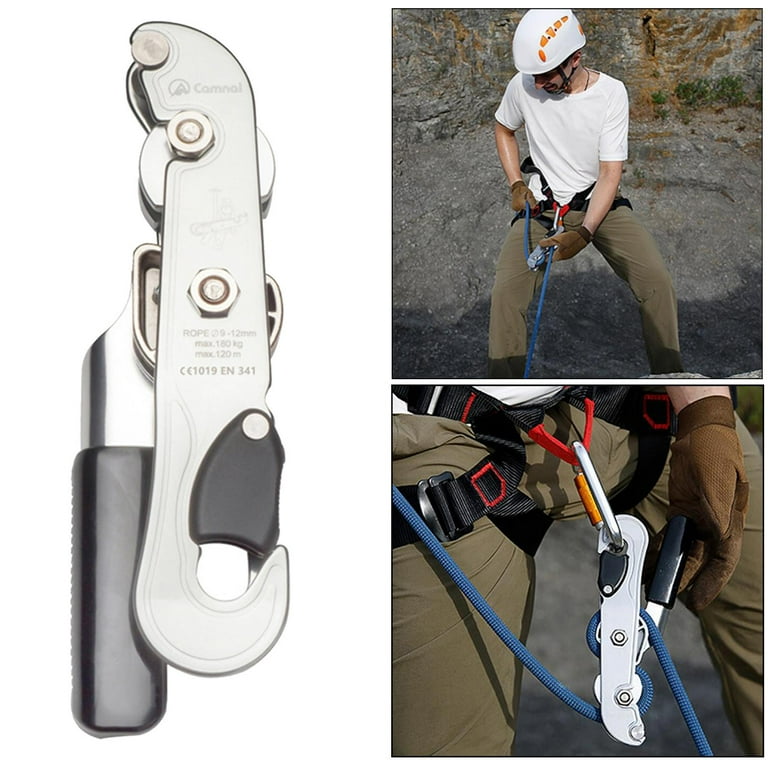The image showcases a piece of climbing gear prominently on the left side, which seems to be used for securing oneself to prevent falls during activities such as rock climbing. The tool, possibly a catapult or a carabiner-type system, features a silver body with a black handle, and has various screws and a clip secured by a black locking mechanism. The background is white, highlighting the tool's design details. Inscribed on the tool are the specifications: "Kamnal, C-A-M-N-A-L, rope, 12 millimeters, max 180 kilograms, max 120 meters, CC1019EN341."

On the right side of the image, two photos illustrate the tool in use. The top photo displays a man dressed in beige pants, a white T-shirt, and a white helmet, equipped with gloves. He is wearing a harness that straps around his waist and legs, connecting to the climbing tool via blue rope and carabiners. The tool is seen central to his waist, aiding in his safety while climbing. The bottom photo provides a close-up view of the man's waist area, detailing the harness and the positioning of the climbing tool with the blue rope threaded through it, demonstrating its practical application in climbing scenarios.